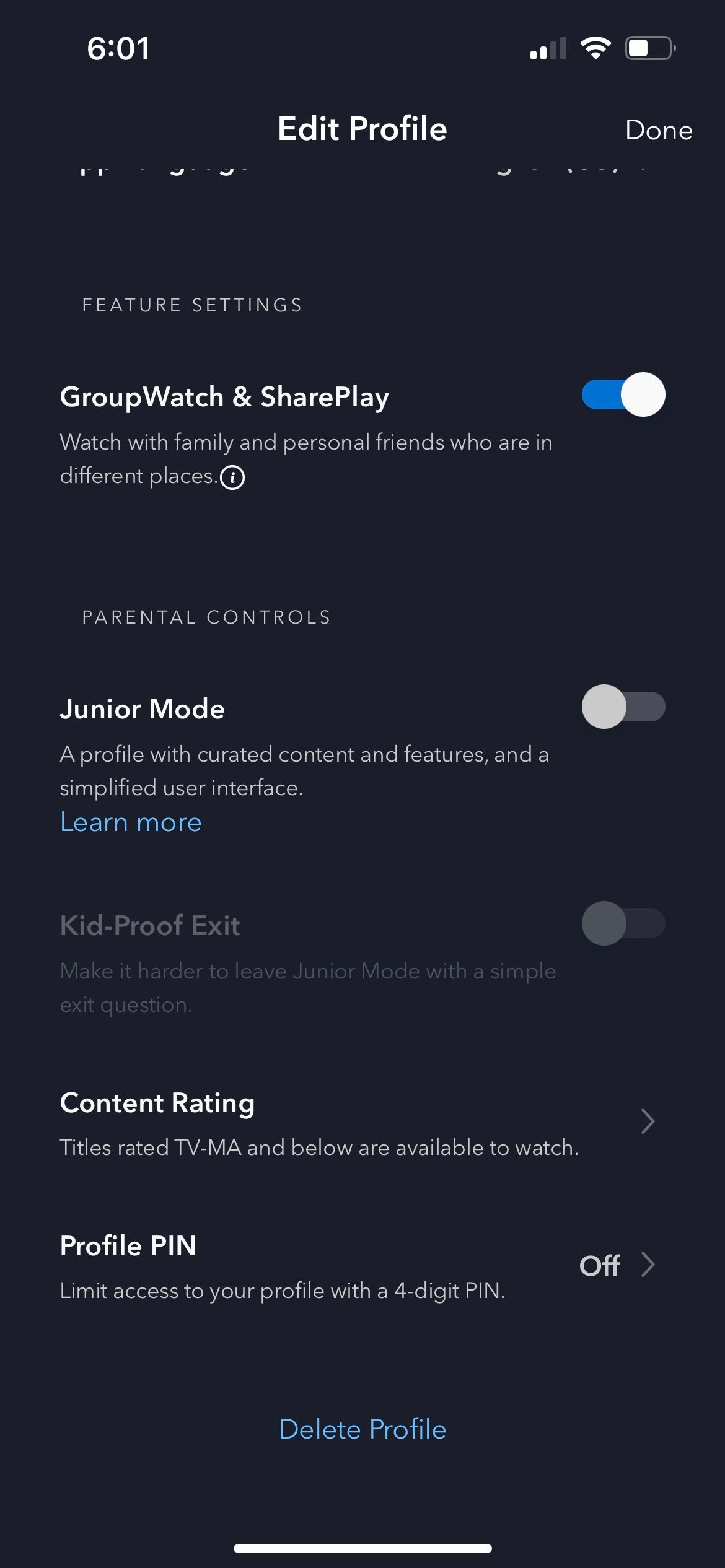Screenshot of a Smartphone Interface

The smartphone screenshot displays a black background with white text, presenting the "Edit Profile" page of an application. The top of the screen shows essential status icons: a Wi-Fi signal indicator, a battery icon at approximately 50%, and a timestamp reading "6:01." 

Below the title "Edit Profile," several features and settings are listed, accompanied by descriptive text and toggle buttons indicating their statuses:

1. **Feature Settings**
   - **Group Watch and Share Play**: Allows users to watch content with family and friends who are in different locations. The toggle button for this feature is blue, indicating it is turned on.
   
2. **Parental Controls**
   - **Junior Mode**: Provides a profile with curated content, features, and an enhanced user interface for younger audiences. The toggle button for this feature is gray, indicating it is turned off.
   - **Kid-Proof Exit**: Adds an additional layer of security, making it harder to exit Junior Mode with a simple question. This feature is also toggled off, with a gray button.

3. **Content Rating**
   - **Titles Rated TV-MA**: Indicates availability of mature-audience content. This section is followed by a right-facing arrow icon.

4. **Profile PIN**
   - **Limit Access**: Allows users to secure their profile with a four-digit PIN. The feature is toggled off, and there is a right-facing arrow icon next to it.

At the bottom of the screen, there is a "Delete Profile" button in sky blue.

The overall interface is designed to provide users with customizable settings to manage content access and profile security efficiently.